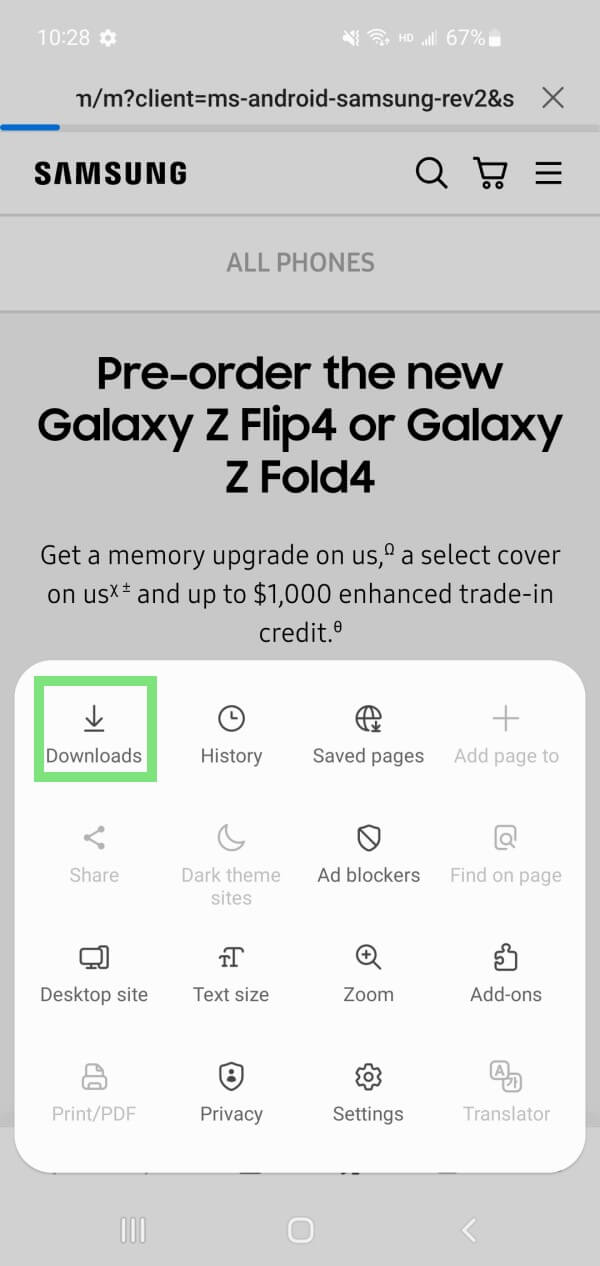The image showcases a variety of UI components against a light purple background at the top. In the top right corner, the time reads "10:28," accompanied by a small white cog icon and a battery indicator showing 67% charge.

Underneath, there's a complex URL string featuring "n/m?client=ms&hash=android_samsung_rev_28 or 2&s," with an adjacent 'X' button. 

Below this, a thin blue line appears, followed by the text "Samsung" flanked by a magnifying glass (search icon) and a shopping cart icon. Further to the right, there are three black horizontal lines.

An advertisement is prominently displayed, announcing: "Pre-order a new Galaxy Z Flip 4 or Galaxy Z Fold 4 to get a memory upgrade on us, plus a select cover included and up to $1,000 enhanced trade-in credit." This message is peppered with various small icons, including circles and 'X' marks for selection or closure.

Near the bottom, a large white box stands out, featuring options in a green-highlighted section for "Downloads." Below this are additional menu items: "History," "Saved Pages," "Add Page As," "Share," "Dark Theme," "Sites," "Ad Blockers," "Find On Page," "Desktop Site," "Text Size," "Zoom," "Add Homes," "Print PDF," "Privacy Settings," and "Translator."

At the very bottom, set against a gray background, there are three more icons: a trio of horizontal lines, a square, and a left-pointing arrow.